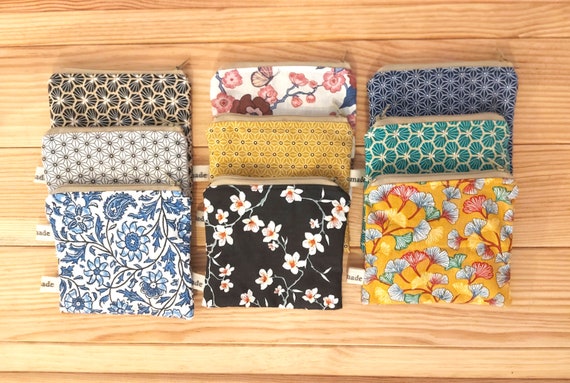On a light-colored wooden table, nine handmade coin purses or makeup bags are meticulously arranged in three rows and three columns. Each purse features a vibrant array of colors and patterns, both floral and geometric, predominantly showcasing hues of black, white, blue, yellow, pink, red, teal, and gold. 

The top row starts with a purse adorned with white and red flowers on a black background, followed by a white one with a red and pink floral motif, and a blue purse with alternating dark blue star patterns. 

In the middle row, the first purse features black fabric with white flowers, followed by a striking gold and white geometric patterned purse, and another purse with a teal background embellished with alternating blue and green lollipop-shaped motifs. 

The bottom row includes a purse with a white background scattered with blue and white flower patterns, another with black fabric showcasing white flowers, and the final purse made from yellow fabric highlighted by pink, blue, and green flowers. Each purse is designed with a zipper top, implying practicality alongside their decorative appeal.